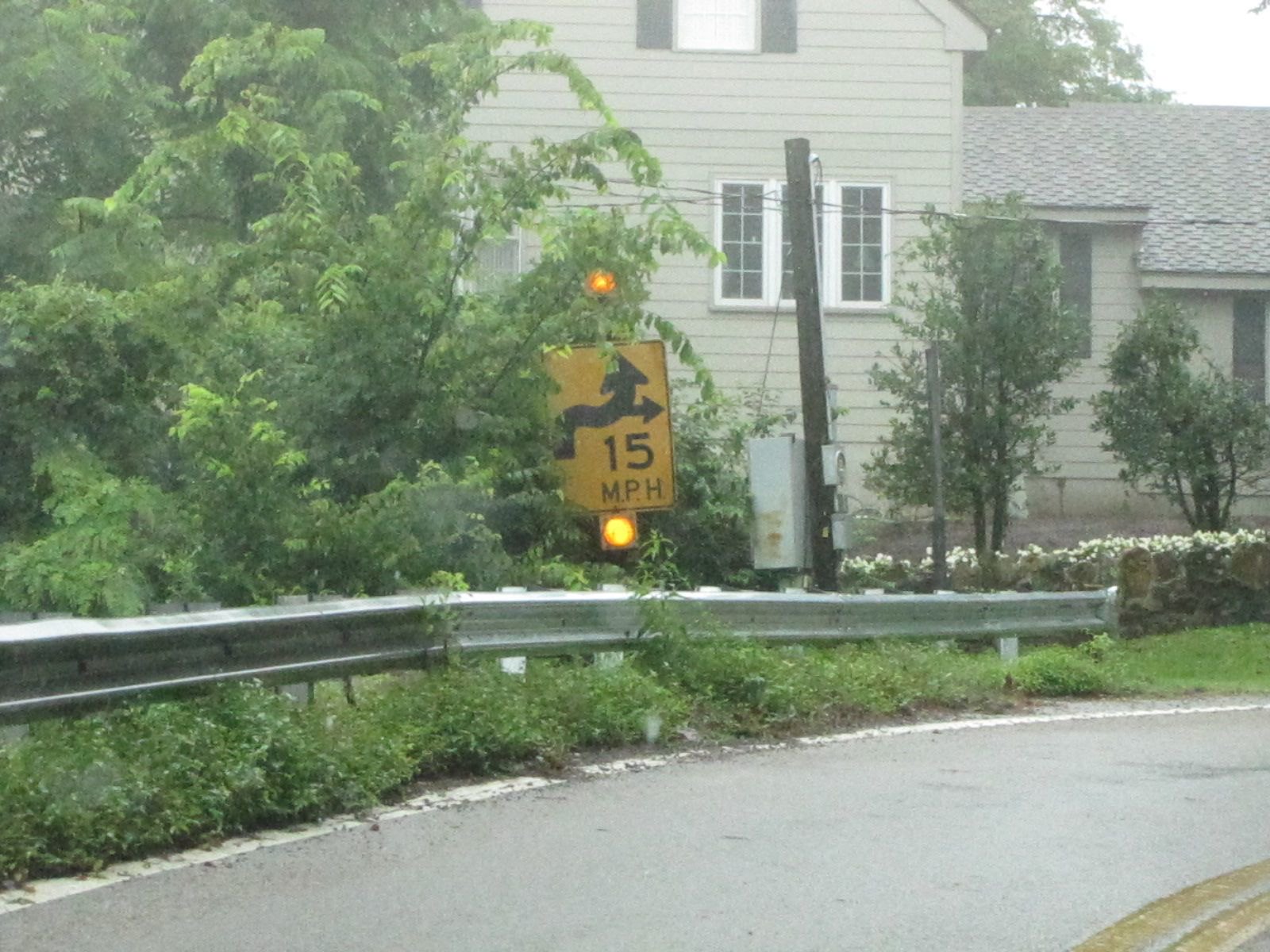This is a detailed color photograph in landscape format, capturing a one-lane road likely designed for one-way traffic. The road curves from the bottom left of the image to the right, bordered by a typical silver or stainless steel guardrail. Dominating the center of the scene is a yellow traffic sign indicating a speed limit of 15 miles per hour and depicting a wavy road. Beneath the sign are two yellow caution lights. Adjacent to the sign on the right, there is a power box and an electric pole with visible power lines extending from it. Behind the guardrail, lush greenery and very light green trees populate the scene, adding an overgrown appearance with weeds, grass, and bushes, some of which have small white flowers. In the distance, a split-level, two-story gray house with wooden paneling and a gray roof is visible. The house has multiple windows, although one is partially obscured by a green tree in front. The surrounding atmosphere appears wet and gray, potentially suggesting a location with frequent rainfall, such as near Portland or Seattle.